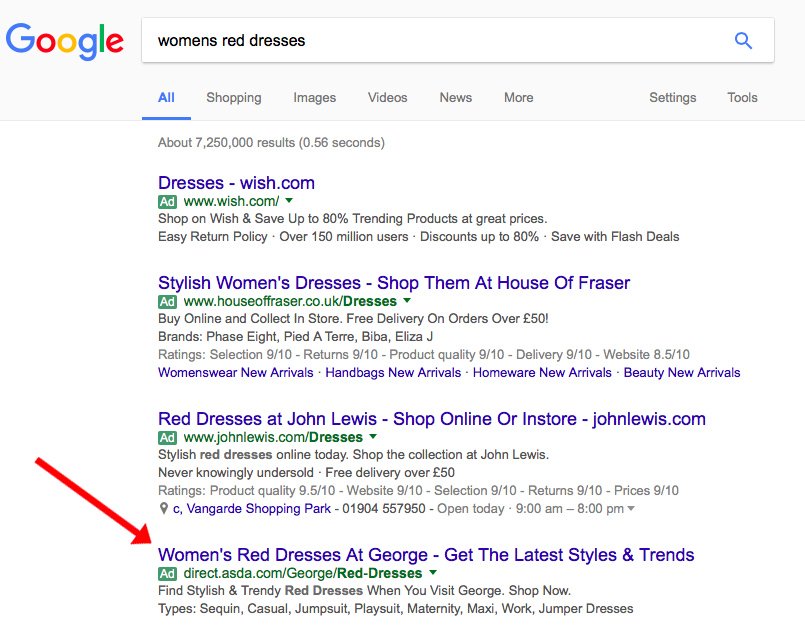The screenshot captures a Google search results page for "women's red dresses." At the top of the screen, the search bar displays relevant query, and beneath it, there are various filter options including All, Shopping, Images, Videos, News, More, Settings, and Tools. The search has yielded over 7 million results, currently set to the "All" filter, displaying primarily links and no images.

The first search result is from Wish.com, highlighting their offer to shop and save up to 80% on trending products. Wish.com touts an easy return policy, a user base of 150 million, and discounts on flash deals, emphasizing their competitive pricing.

The second result comes from House of Fraser, a UK-based retailer, promoting stylish women's dresses. The description mentions options to shop online and collect in-store with free delivery on orders over £50. They carry brands such as Phase Eight, Petite, Biba, and Eliza J. The store boasts high ratings with a 9 out of 10 for selection, returns, product quality, and delivery, and an 8.5 for website usability. Additional specifics can be explored by clicking on various links.

Further down, there's a mention of red dresses available at John Lewis, followed by a listing for women's red dresses at George, associated with Asda.com, which promises the latest styles and trends.

Overall, this detailed search results page offers various options for users looking to buy women's red dresses from different retailers.